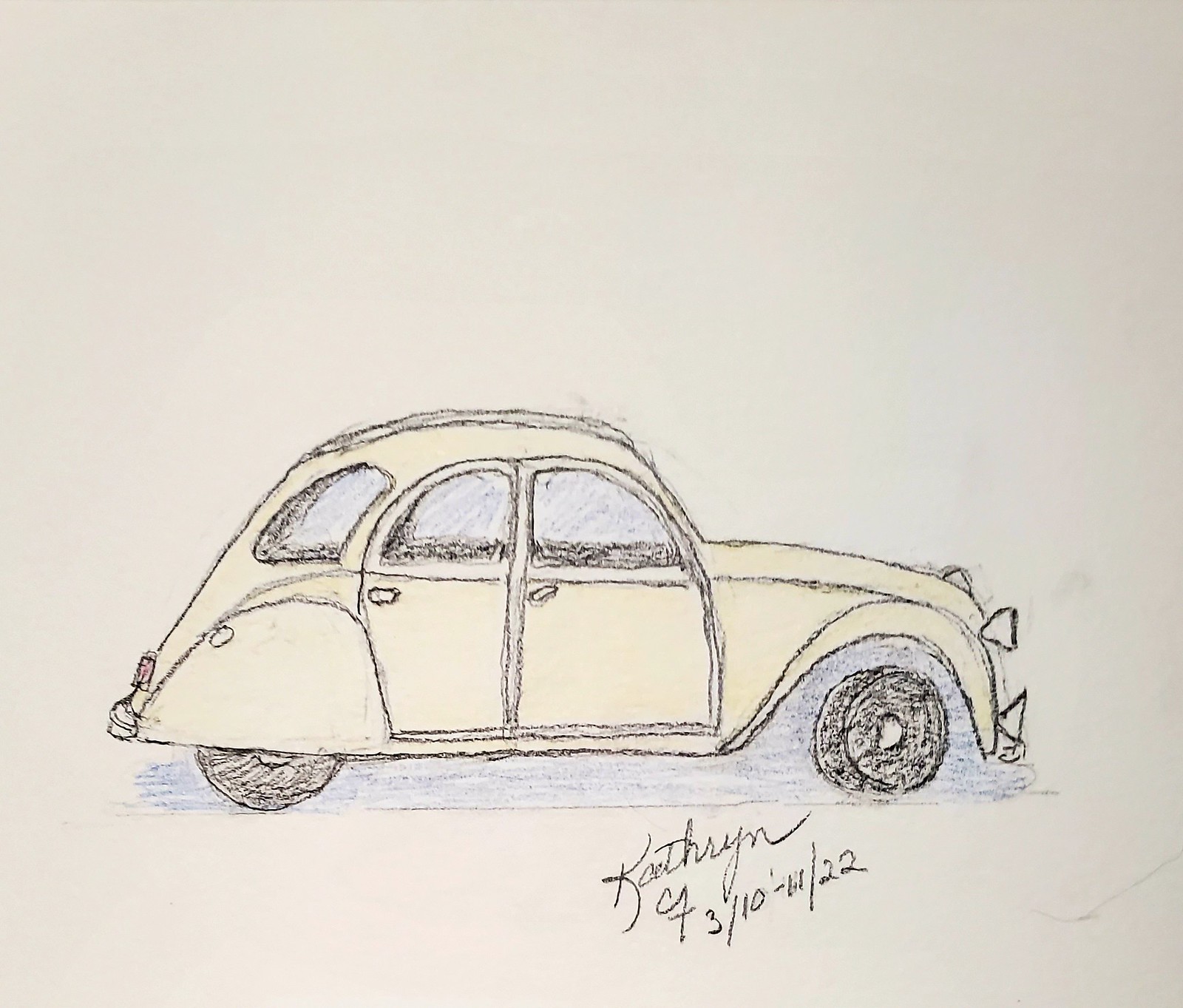This side-view colored pencil drawing depicts a vintage-style vehicle closely resembling a Volkswagen Beetle but with distinct modifications. The car features a longer hood and four doors, maintaining the classic rounded dome shape iconic to the Beetle. Rendered in a soft pale yellow hue, the car's structure is defined with precise dark pencil outlines. A subtle blue shadow lies beneath the vehicle, adding depth to the illustration. The tires are shaded black, complementing the car's classic aesthetic. Attention to detail is evident with the inclusion of a tail light, a license plate, headlight, and a double bumper setup—both at the front and rear. The artist has signed the piece at the bottom: "Catherine F, 3/10-11/22."